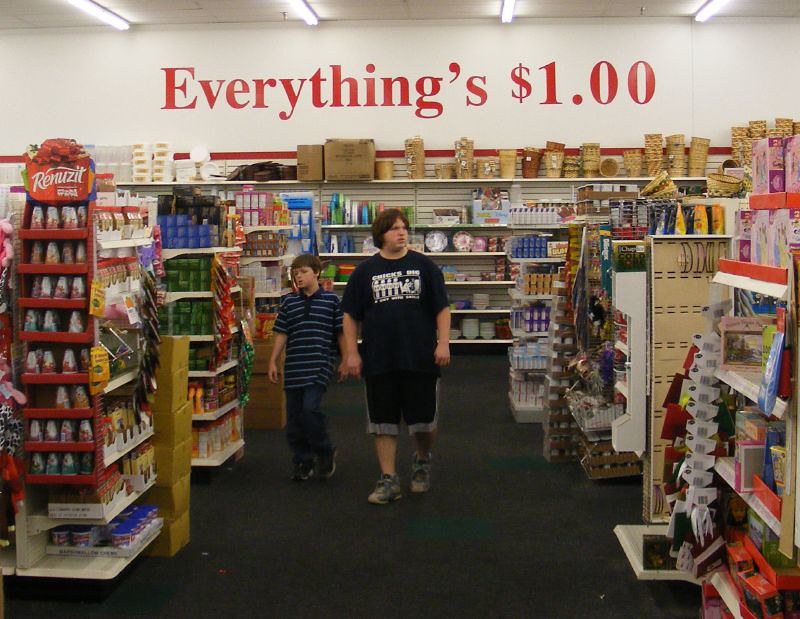The image captures the bustling central aisle of a dollar store. At the very top of the photograph, a large red sign boldly proclaims, "Everything's One Dollar," immediately drawing attention. Above this sign, four fluorescent lights partially peek out, casting a quintessential dollar store glow over the scene. Below the prominent sign, the back shelves are lined with a variety of items, including plant pots, possible bottles of shampoo and conditioner, and other assorted household goods. 

In the middle of the aisle, walking towards the camera, are two young boys. The older boy appears to be around 14 or 15 years old. He is dressed in a black t-shirt adorned with white writing, black shorts, and grey running shoes. Beside him is a younger boy, likely his brother, who looks to be about 10 or 11 years old. He is wearing an oversized blue polo shirt with white stripes, buttoned up completely—a probable hand-me-down from his older sibling. His outfit is completed with blue jeans and black shoes.

On either side of the boys, the aisle ends display small arrangements of products, and other various items fill the shelves, each marked with the allure of being priced at just one dollar. This visual encapsulates the typical dollar store atmosphere, bustling with affordable everyday essentials and multiple bargains.